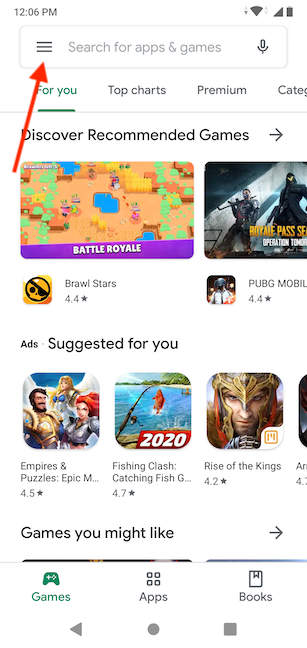This is a detailed screenshot of an Android device displaying a game or app store interface. At the top, there is a prominent search bar containing the placeholder text "Search for apps & games." Within the search bar's confines, a red arrow, likely overlaid on this image, points at a hamburger button. To the right of the search bar, a Google system UI microphone icon allows for voice searches.

Directly below the search bar is a horizontal tab for navigation, featuring options like "For You," "Top Charts," "Premium," and partially visible "Categories." Underneath this tab, the heading "Discover Recommended Games" is accompanied by a right-pointing arrow, indicating more content available with scrolling.

In the visible section of recommended games, the first game highlighted is "Brawl Stars," displayed with a screenshot featuring a Battle Royale scene against a purple background. The game boasts a 4.4 rating. To the right of "Brawl Stars," part of the listing for "PUBG Mobile" is visible, though only half of the screen is shown, suggesting more content available upon scrolling.

Further down, there is an ad section titled "Suggested For You," showcasing colorful icons for games such as "Empires & Puzzles," "Fishing Clash," and "Rise of the Kings." Another partially visible section, "Games You Might Like," is also present, though its contents are obscured.

At the bottom of the screen, a navigation bar displays three tabs: "Games" (currently selected and highlighted in green), "Apps," and "Books," representing different sections of the store. Below these tabs, familiar Google UI elements provide standard navigation options throughout the user interface.